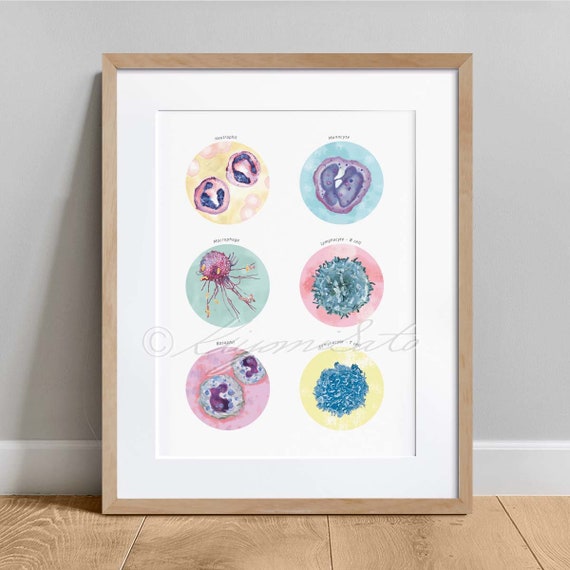This image features a striking piece of art depicting six colorful, circular microbiology-inspired designs, framed with a light pine or maple wood color and accented by a white matte. The frame, leaning against a bland gray wall, is set on a hardwood or bamboo-type light brown floor. Each circle showcases a different pastel-colored, magnified cell-like structure. The top left circle combines pink, blue, and yellow hues, featuring pink orbs with blue interiors against a yellow backdrop. The top right circle has an ocean-blue background with a central red-purple blob speckled with blue and pink. The middle left circle could resemble a flower, displaying a teal background with a pink flower-like structure. The middle right circle features a blue circular 'furball' on a pink background. The bottom left circle shows a pink background with two large blue circles, each containing purple and smaller blue orbs inside. The bottom right circle presents a lime green background with another blue hairy circle. A copyright mark, possibly spelling "Kinomisato," is visible on the photo, adding an element of authenticity to the artwork.